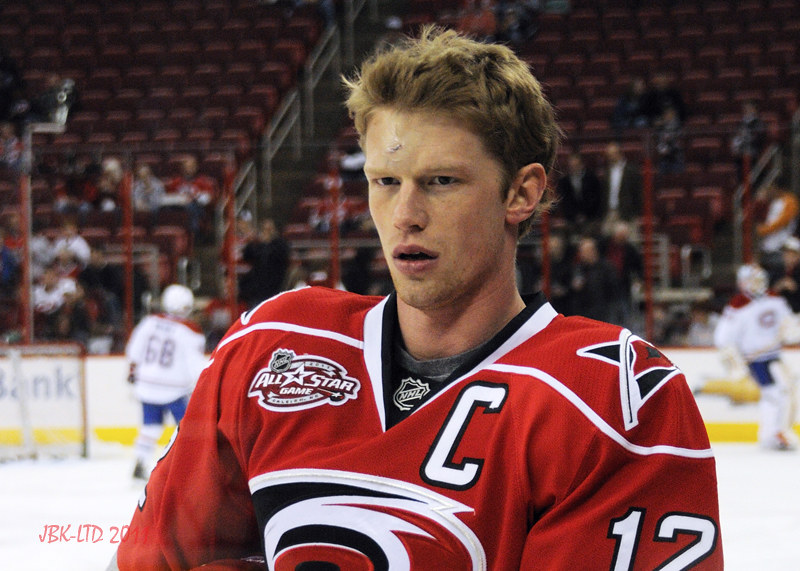In this detailed close-up image of an NHL hockey player, the focus is on a young man with brown hair and a serious expression, dressed in a red jersey with the number 12 barely visible. He wears a black undershirt emblazoned with an NHL logo, denoting his participation in an All-Star game—further emphasized by the All-Star logo featuring a star and the NHL emblem on his right shoulder. As the team captain, a white "C" is prominently displayed on the left side of his chest. The jersey also includes a distinct red, black, and white swirling logo, akin to the Carolina Hurricanes’ emblem. Behind him, within the ice rink, are additional hockey players in white jerseys with blue pants and white helmets, including one facing away with the number 66. The arena background reveals the ice, rink walls, and stands with a smattering of spectators amid mostly empty red seats.